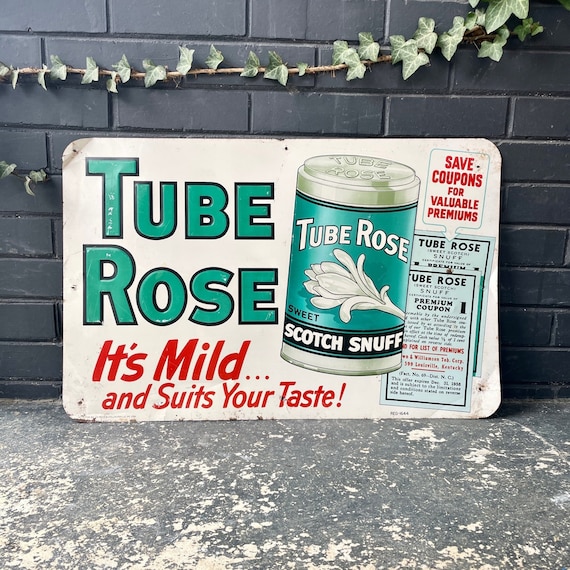The image features an old-fashioned metal advertisement sign, prominently displayed against a dark gray bricked wall, partially covered with ivy. The sign itself, with a white background, is leaned up against a speckled, dark gray sidewalk. Centered at the top of the sign, the text "Tube Rose" is shown in a teal green font, with the red text below it stating, "It’s mild and suits your taste." A depiction of a canister labeled "Tube Rose Scotch Snuff" with a white flower silhouette is also visible. To the right of the canister, there are illustrations of two pieces of paper with text, one of which reads, "Save coupons for valuable premiums" in red font. The floor beneath the sign has a distinctive pattern of white speckles amid the dark gray, further highlighting the aged and nostalgic appearance of the scene.